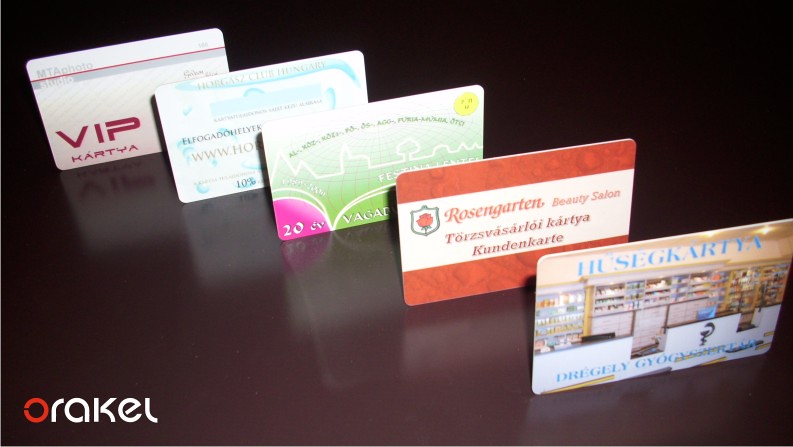In this vibrant color photograph, five neatly arranged credit card-sized items, likely gift or membership cards, are prominently displayed on a very dark brown tabletop, contrasting sharply with the background. The cards are not lying flat but appear to be standing upright, possibly supported by an unseen mechanism. Dominating the lower left corner, the word "Oracle" is distinctly written with a red 'O' followed by 'RAKEL' in white. The cards are positioned in a slightly zigzag manner, adding a dynamic visual flair. 

The first card, labeled "VIP MTA Photos," appears designed for frequent users of a particular service. The second card partially reveals a web address ending in "club hungry," suggesting a loyalty or discount program. The third card, a striking lime green, boldly features the number twenty. The fourth card, in red and white, advertises the "Rosengarten Beauty Salon." The final card, marked "Huskyardia," remains somewhat mysterious. This captivating arrangement and the precise detailing point toward a meticulously crafted advertisement.